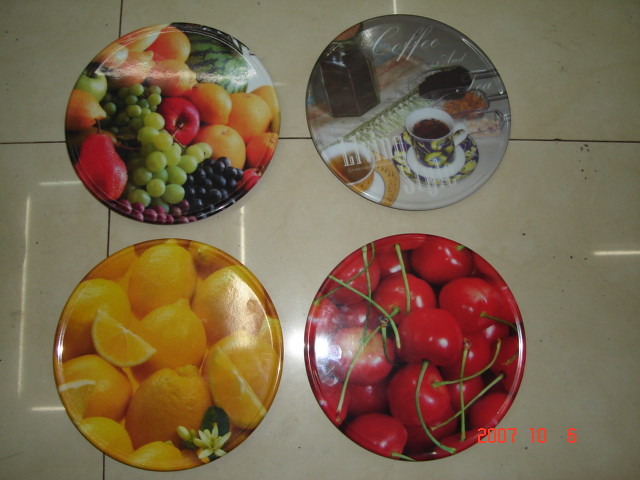This image depicts four circular plates arranged on a white tiled surface, possibly a floor or table, with the date "2007-10-6" displayed in the bottom right corner. Each plate features a distinct and vibrant design. The top left plate showcases a variety of fruits, including pears, apples, oranges, green and purple grapes, and a slice of watermelon. The top right plate is dedicated to coffee and tea, featuring a cup of coffee, a jar possibly containing coffee beans, and the words "coffee and living" engraved on it. The bottom left plate displays several cut lemons, while the bottom right plate is filled with cherries. The white tiled background appears to be either formica or a marbled surface, though it's challenging to determine if the plates are hanging on a wall or lying flat.